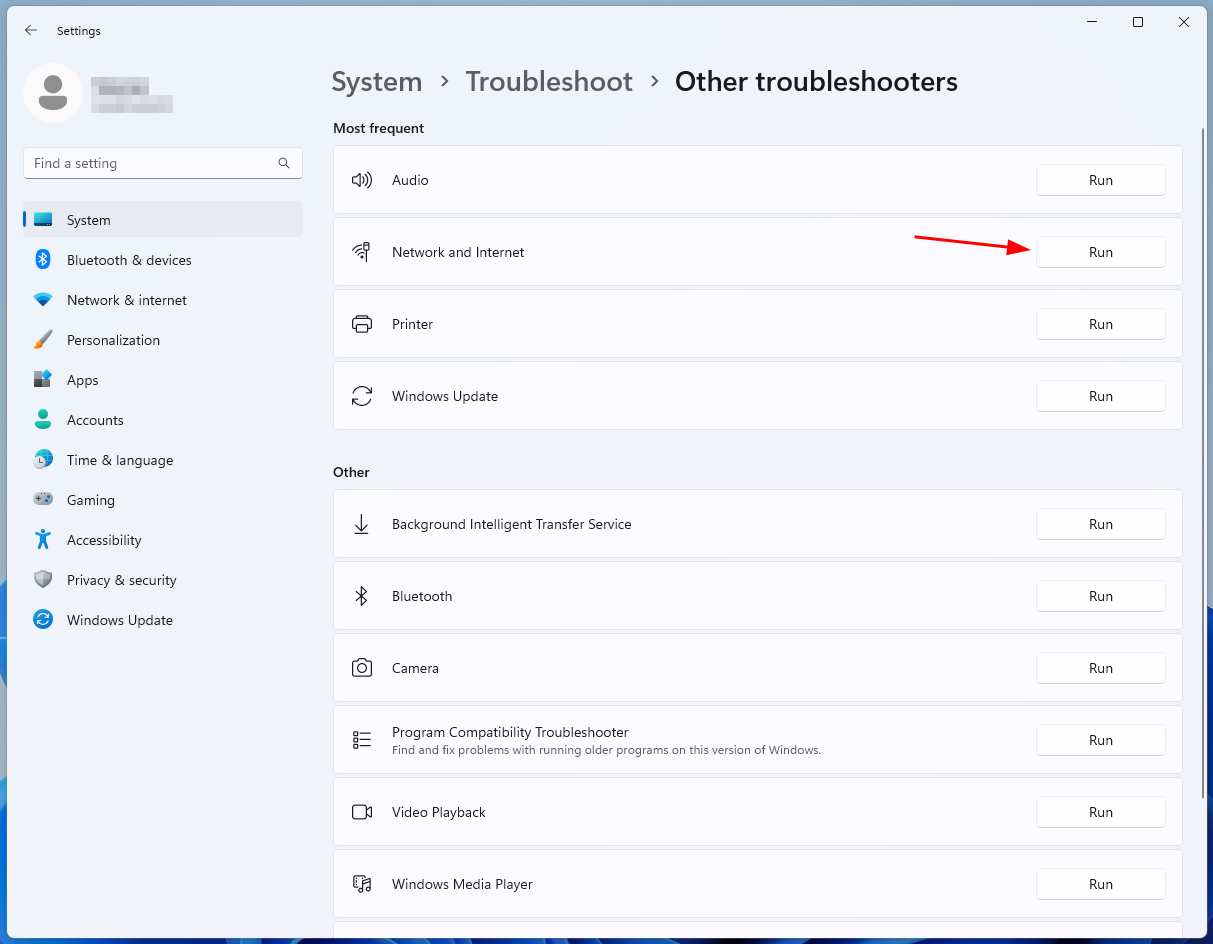The image is a screenshot of a settings section, likely from an app or a website, focused on troubleshooting options. At the top of the page, there are categories labeled "System" with a right arrow pointing to "Troubleshoot" and another arrow leading to "Other troubleshooters." The first section, titled "Most frequent," lists common troubleshooting options including:

1. Audio
2. Network and Internet
3. Printer
4. Windows Update

Each of these options has a white "Run" button positioned on the right side. Notably, there is a red arrow pointing towards the "Run" button next to the "Network and Internet" option. The arrow's tip touches the button's box, and its tail extends towards the upper left quadrant.

The subsequent section is labeled "Other," listing additional troubleshooting categories such as:

1. Bluetooth
2. Background Intelligent Transfer Service
3. Camera
4. Program Compatibility Troubleshooter
5. Video Playback
6. Windows Media Player